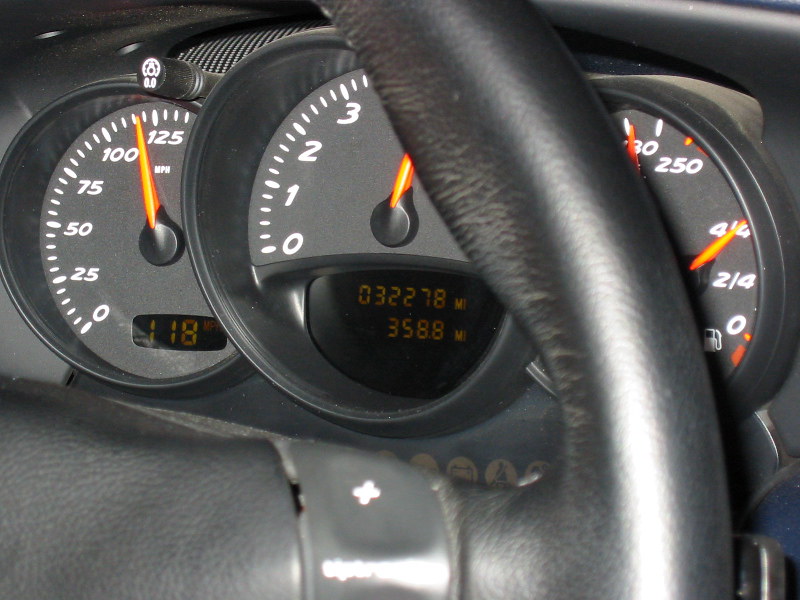The image displays the dashboard of a vehicle, likely a Mazda, based on the distinct text font style used in the instrument panel. On the left side, the speedometer is marked in increments from 0 to 125 miles per hour, currently indicating a speed of approximately 120 mph, suggesting the vehicle is traveling at a high speed.

Centrally, there is a tachometer that measures the engine's revolutions per minute (RPM), graduated from 0 to, presumably, around 8, though only up to 4 is visible due to the steering wheel partially obscuring the gauge. Adjacent to the tachometer, there is a fuel gauge showing a full tank.

To the right, another speedometer, likely part of a secondary or more detailed display, is visible and marked up to 250 mph, though it is mostly obscured in the image. The odometer reading indicates the vehicle has traveled 3,222 miles, additionally displaying the trip mileage as 358.8 miles.

The dashboard and steering wheel are black, contributing to a sleek, modern interior aesthetic typical of Mazda's design language.